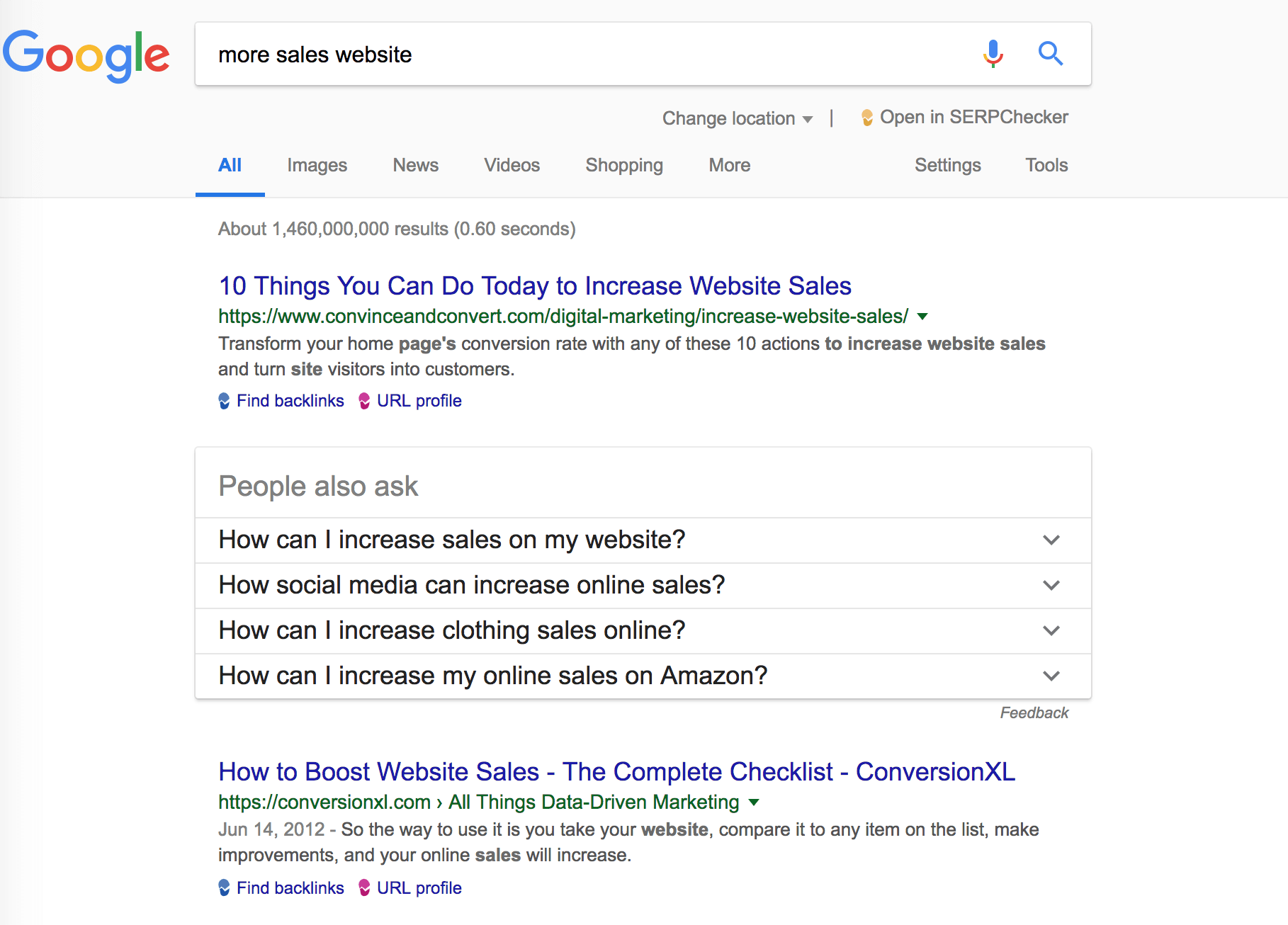The image depicts a Google search results page. In the upper left corner, the recognizable Google logo is present, accompanied by a search box containing the query "more sales website." Just below, navigation options such as "Change location," "Open Insert Checker," and others like "All," "Images," "News," "Videos," "Shopping," and "More" can be seen, along with "Settings" and "Tools" options. The search yielded approximately 1,460,000,000 results within 0.60 seconds.

Prominently displayed is a result from the website www.convinceandconvert.com under the path /digital-marketing/increase-website-sales/. The webpage's title reads, "10 Things You Can Do Today to Increase Website Sales," with the description promising to help transform your homepage's conversion rate with actionable tips to turn site visitors into customers.

Further down, a section labeled "People also ask" presents popular queries such as:
- How can I increase sales on my website?
- How can social media increase online sales?
- How can I increase clothing sales online?
- How can I increase my online sales on Amazon?

Additional details below this are also visible, though not specified in this description.